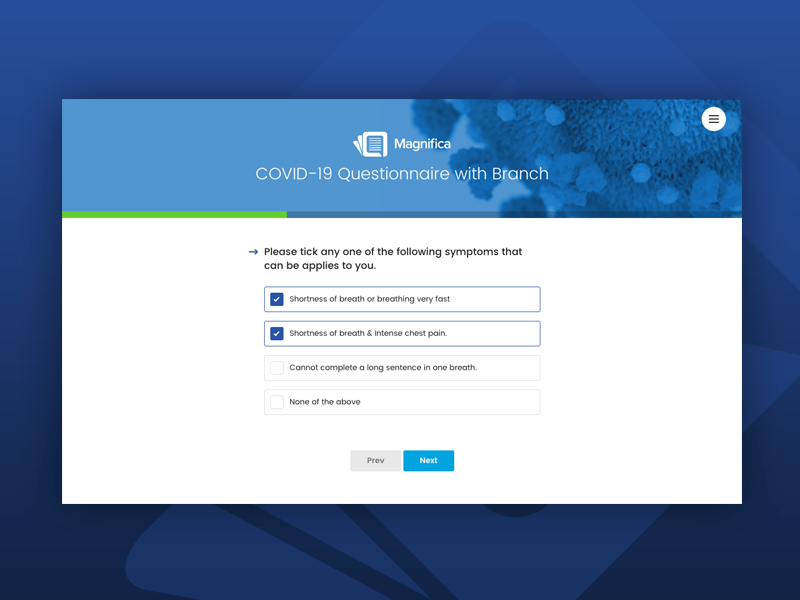This image is a screenshot of a questionnaire page hosted on a website. The overall background features a dark and light blue angular pattern that adds a modern, dynamic feel. Floating above this pattern is a primarily white screen with a blue header, casting a faint shadow on the backdrop.

At the top of the white screen is a vivid blue header. On the right side of the header, there is an artist's impression of a Vyron, tinted in shades of blue. The center of the header reads "Magnifica COVID-19 Questionnaire with Branch" in clear, bold text. Positioned in the top right corner of this header is a circular white menu button featuring three horizontal gray lines.

Directly beneath the header lies a thin green progress bar. This bar is filled about a quarter of the way and continues in a translucent blue that overlays part of the blue header.

Within the white area of the screen, a question prompts the user: "Please tick any one of the following symptoms that apply to you: Sick." Below this inquiry are four checkbox options:
1. "Shortness of breath or breathing very fast" – This option is selected, indicated by a blue box with a white checkmark surrounded by a blue line.
2. "Shortness of breath and intense chest pain" – This option remains unchecked.
3. "Cannot complete a long sentence in one breath" – This option is also unchecked.
4. "None of the above" – This option remains unchecked as well.

At the bottom of the screen are navigational buttons. The left button is gray and labeled "Prev," while the right button is blue, labeled "Next" in white text.